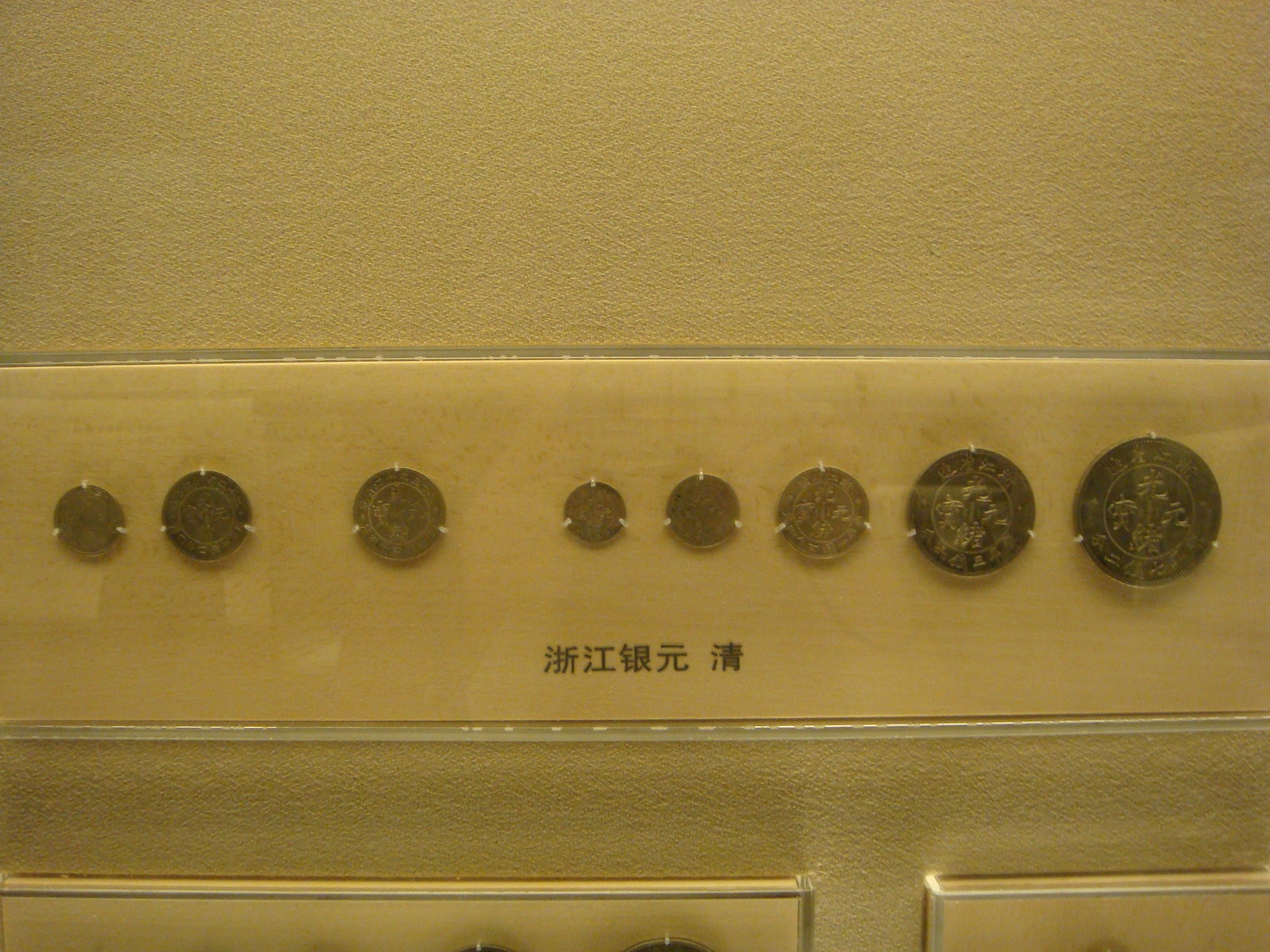The image showcases a striking collection of coins displayed against a gold-colored backdrop. Prominently featured at the center of the photo are eight coins of varying sizes, secured horizontally in a clear case. Distinctly marked with Chinese writing, the coins—ranging in size from that of an American penny to an American dollar—add an exotic flair, suggesting they are likely of Chinese origin. Each coin is meticulously sewn into place with three white threads that hold them against a beige background, which seamlessly transitions into a beige wall, implying that the display might be part of a museum exhibit or a private collection. The clear casing houses the coins with no visible reflections, adding to the enigma of the setting. Below these primary coins, there appears to be tips of additional coins in other cases, hinting at an extensive collection. The structured arrangement, along with the detailed inscriptions on the coins, blend the essence of historical preservation with an aesthetic display.